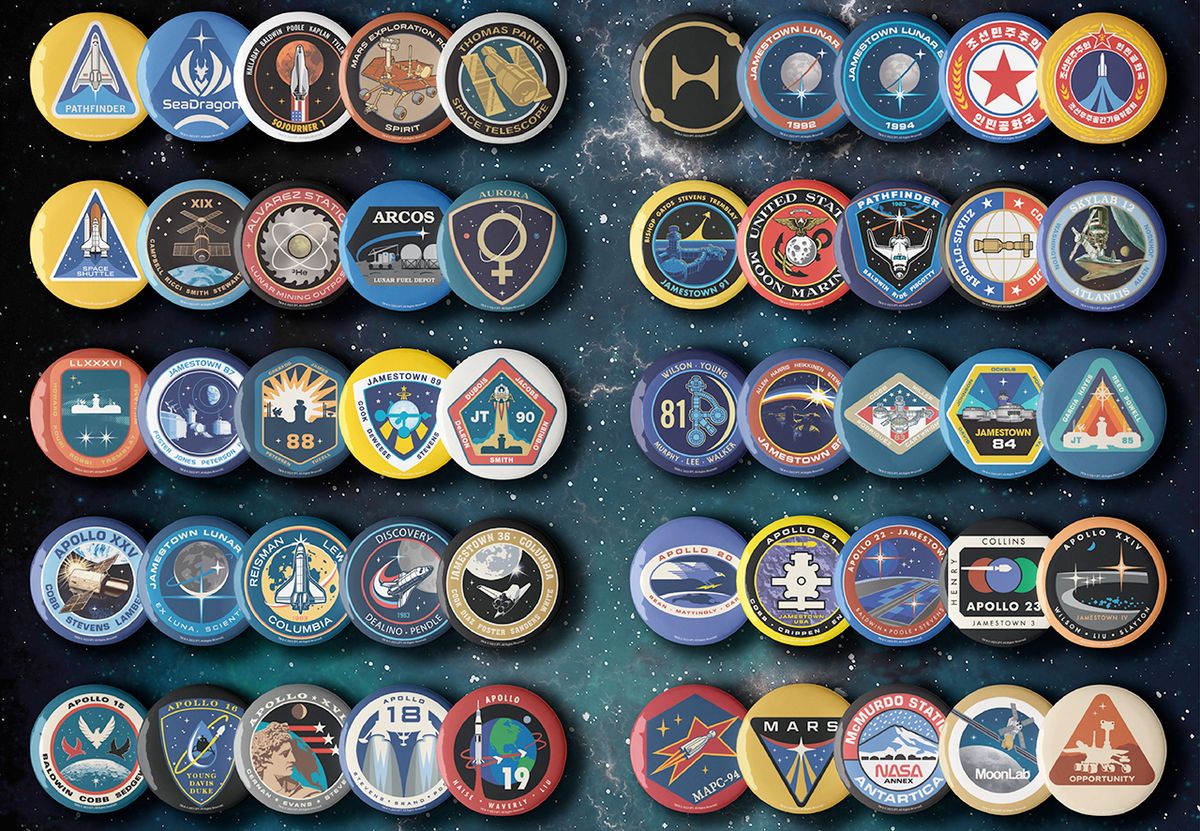The image displays a meticulously arranged compilation of 50 colorful and diverse space-themed badges or patches, organized into five rows with ten patches each. The badges, primarily related to various space programs, prominently feature spaceships, planetary imagery, and names like Apollo 15, Discovery, Pathfinder, Jamestown, and Opportunity. Each badge is distinct, vividly illustrating different space missions and exploration endeavors. The patches are separated in the center, creating distinct groups of five-by-five. The background of the image enhances the space theme, depicting a stunning night sky filled with stars and nebulae, creating a celestial ambiance that complements the details on the badges.